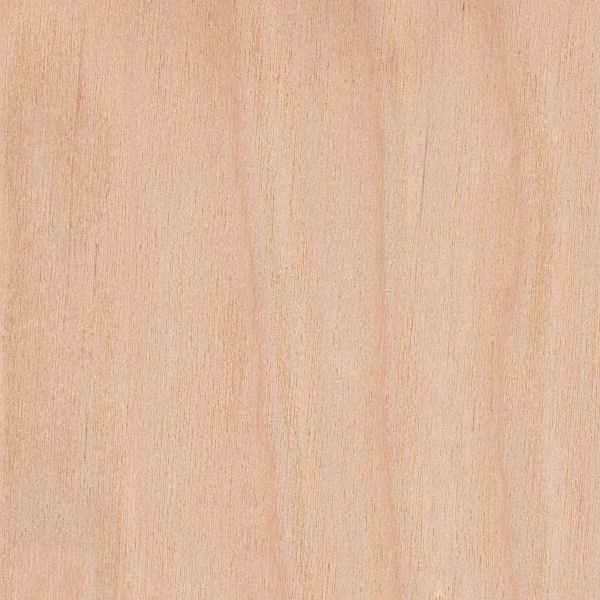The photograph depicts a rectangular wooden countertop made of light, pale brown pressed plywood, typical of the kind you might find in a school setting. The surface is a single, uninterrupted sheet rather than separate planks or boards, featuring a natural color with visible grain lines and minor imperfections. A tiny black mark is noticeable towards the top, and the wood shows slight variations in coloration, reminiscent of school desks commonly found in biology, English, or health classes.